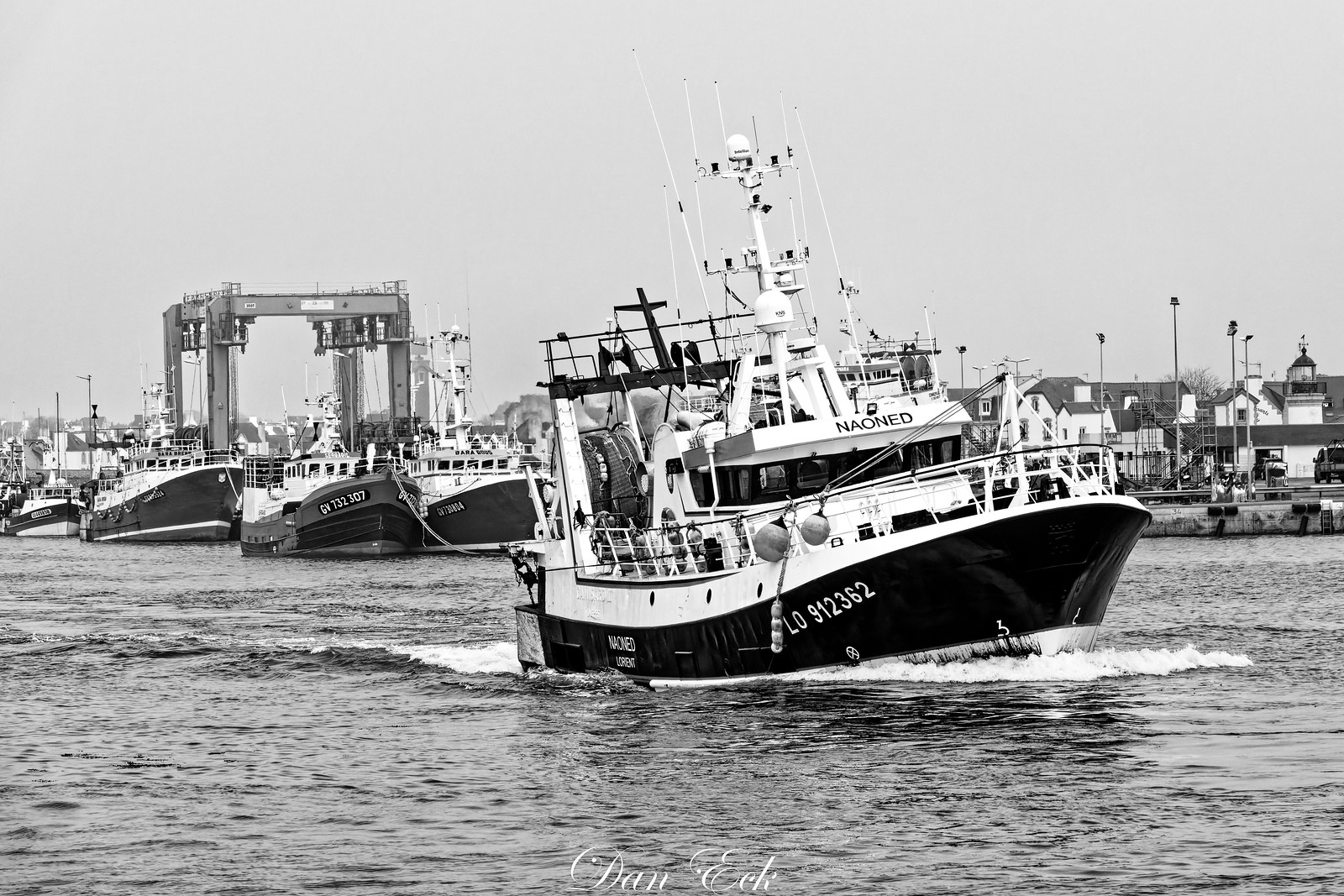The black and white photograph captures a dynamic scene on the water, featuring a prominent black boat with white trim at the center. The boat, identified by the name "NAONED" and the ID number "LO912362" on its hull, is moving through the water, creating white cresting waves beneath it. The lower part of the boat bears the name "Dan Eck" in white letters. Above the cabin, sophisticated navigation equipment is visible, suggesting it is a well-equipped and maneuverable vessel, possibly used by the Coast Guard or for towing. The backdrop reveals a marina with multiple stationary boats docked, and an array of houses and buildings lining the horizon under a gray, overcast sky. Additionally, a large boat lift, capable of hoisting sizable yachts, is discernible in the far background, adding depth to the overall maritime setting.